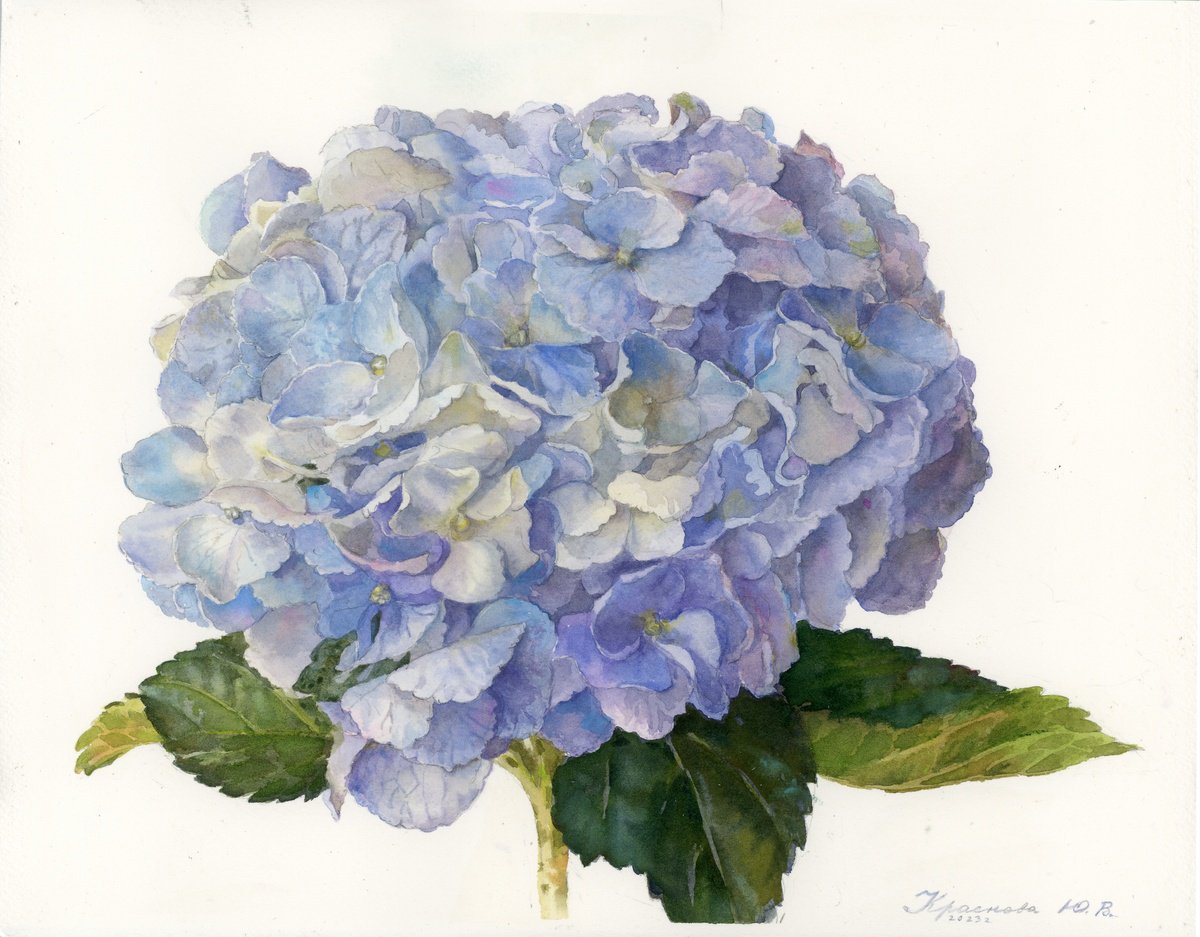This image showcases a detailed watercolor painting of a bouquet of various blue and purple flowers, all stemming from a single light green stalk. Dominant colors include shades of blue—ranging from light blue to indigo—and vibrant purples with touches of violet. Additionally, there are accents of green and light yellow, particularly in the leaves and the centers of some flowers. The flowers, clustered together in a vivid, puffy arrangement, display a delicate blend of petals, some with pale yellow or whitish centers, contributing to their intricate and whimsical appearance. The painting's background is kept minimalist, a pristine white, which further emphasizes the rich hues and intricate details of the floral bouquet. In the bottom right corner, the artist's signature, which includes discernible letters like "K," "P," and "A," along with a date "2023," is inscribed, adding a touch of authenticity and personal touch to the artwork.